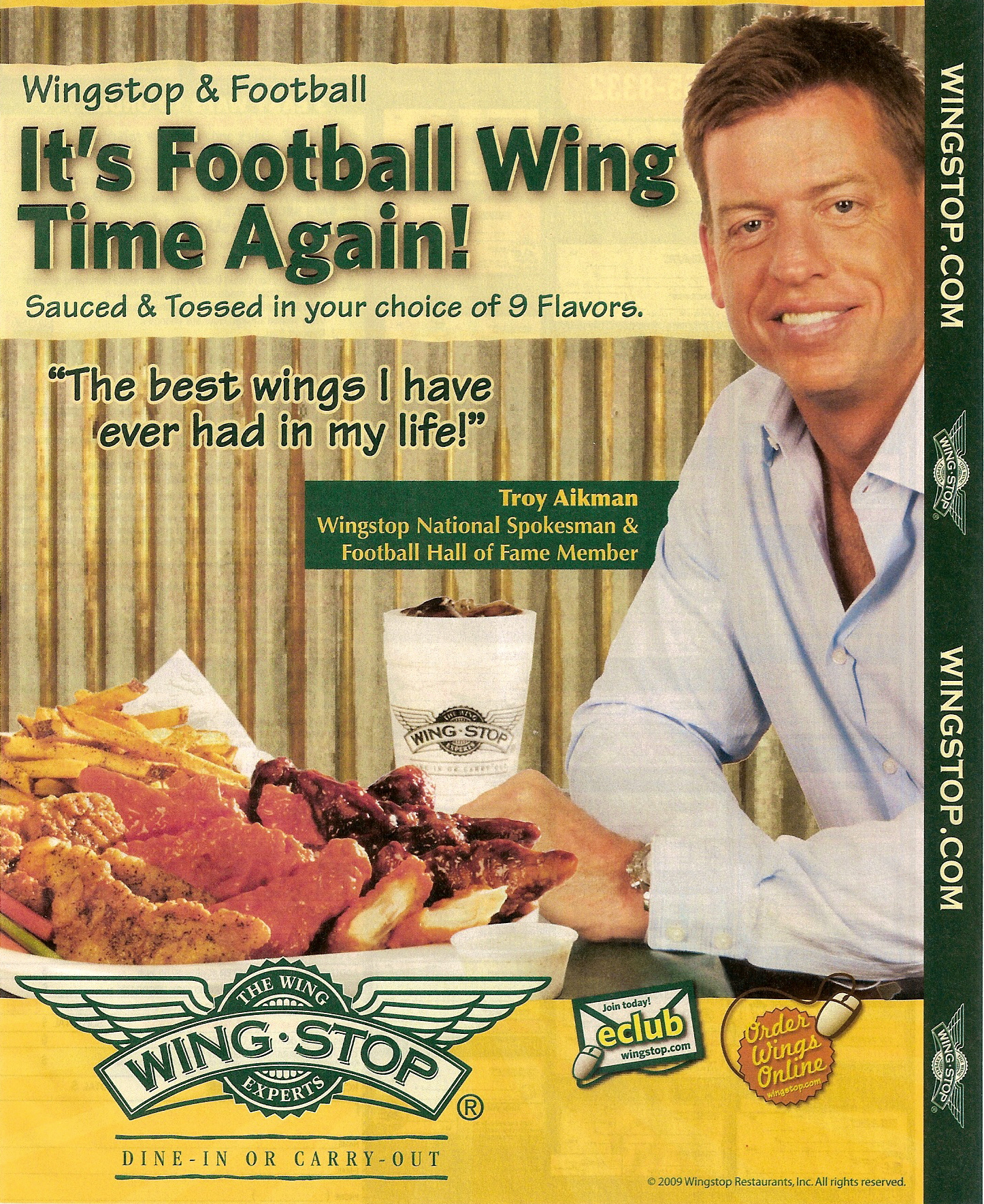This image is a detailed advertisement for Wingstop, featuring a photograph of Troy Aikman, the Wingstop National Spokesman and Football Hall of Fame member. The background is brown and white striped, with a prominent tan box at the top containing green, bold text that reads, "Wingstop and Football: It's Football Wing Time Again!" followed by the phrase, "Sauced and tossed in your choice of nine flavors." Positioned at a table, Troy Aikman sits smiling, dressed in a white button-down shirt. His arms are folded on the table, and he holds a Wingstop-branded cup likely containing Pepsi. In front of him, there's a large bowl filled with an assortment of chicken wings and french fries.

Adjacent to Troy Aikman, text in a green box with yellow letters states, "Troy Aikman: Wingstop National Spokesman and Football Hall of Fame Member." Below this, additional text reads, "The best wings I have ever had in my life." The Wingstop emblem, resembling airplane wings, is prominently placed with the tagline "The Wing Experts." Instructions for "Dine In or Carry Out," along with promotions for the E-Club and ordering wings online, are featured. It also includes vertical text on the right-hand side that says "wingstop.com" twice, with a green background, reinforcing the web address for further engagement.